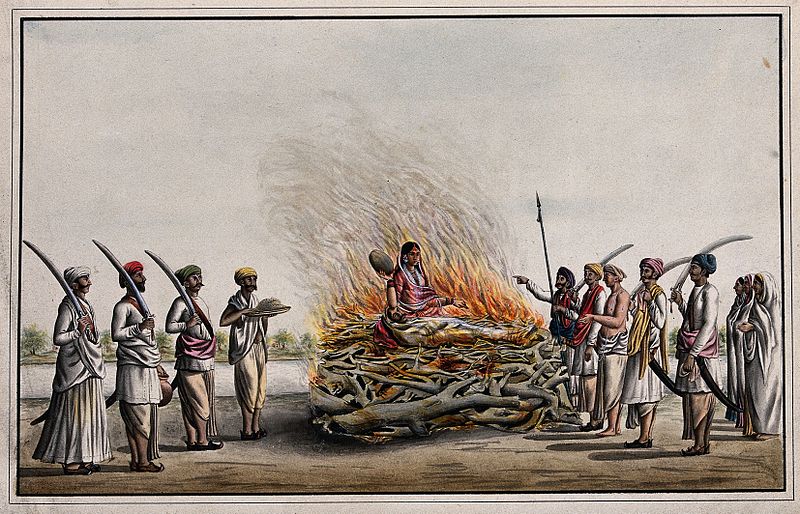The painting depicts an ancient Indian ritual, possibly sati, where a woman, dressed in a vibrant red sari with a pink dot on her forehead, sits solemnly on a burning pyre next to the shrouded body of her deceased husband. Above the heap of wood, flames rise in shades of yellow and orange, casting a solemn glow. Surrounding this central scene, men and women stand solemnly, many men holding swords, some clad in white garments while others sport more colorful attire. The ground beneath them is a parched brown, and the sky overhead is a somber gray, enhancing the grim atmosphere. The painting itself is enclosed with a repetitious black border, adding to the gravity of the scene depicted.